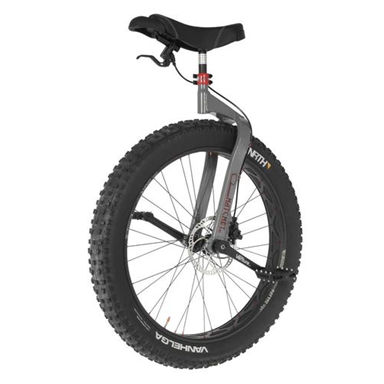The image showcases a modern unicycle set against a pristine white background that seamlessly blends with the edges, enhancing the focus on the product. The unicycle features a robust, black, all-terrain tire embellished with the name brand "Van Helga" in white script along its sidewall. This tire, characterized by its deep ridges and thick profile, seems tailored for challenging environments such as snow or water.

The unicycle's structure is fortified by a silver frame adorned with metallic spokes that radiate from the central axle. It stands on two entirely black pedals equipped with spikes to ensure secure footing. Extending above the tire, the silver frame supports a strong neck leading up to a black bike seat. Beneath the seat, a red band punctuated by a white strip adds a touch of color contrast.

A distinctive feature of this unicycle is the integrated handbrake system, cleverly positioned under the seat with its wire running discreetly down to the tire, offering advanced control and safety for the rider. This unicycle marries rugged functionality with modern design, making it a unique and visually appealing mode of transport.